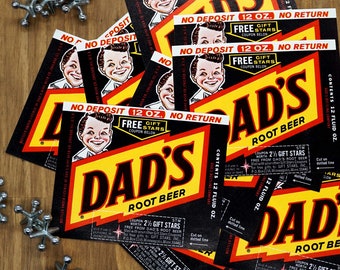The image showcases a close-up, bird's-eye view of a wooden table scattered with approximately eight to thirteen labels from Dad’s Root Beer bottles. These labels dominate the center and right side of the dark brown wooden surface, partially obscuring one another. Each label is square with a distinct yellow polygon in the center bearing the black text "Dad's Root Beer." Across the top of each label, in red letters on a white background, are the phrases "No Deposit," "12 Ounces," and "No Return." The labels also feature a cartoon image of a man's face in the top left corner and additional finer print around the edges. Additionally, small metal jacks, typically used in the game of jacks, are positioned in the bottom and top left corners of the table, adding a nostalgic touch to the scene.